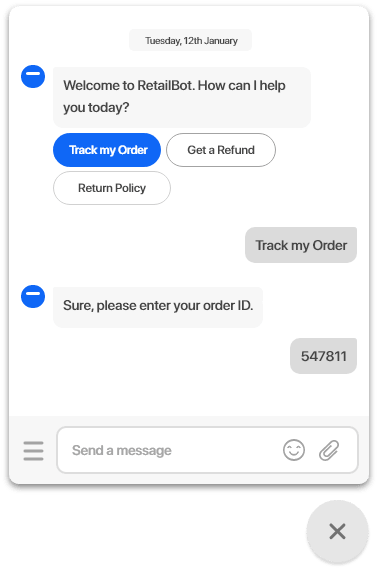**Detailed Caption:**

The image showcases a screenshot of a chat interface between a user and a chatbot, enclosed within a sleek rectangle with curved corners, accentuated by a soft shadow. Centered at the top on a white background is a light gray rectangle bearing black text that reads "Tuesday, 12th January."

The conversation begins with the chatbot, represented on the left side by a blue circular avatar featuring a white dash at the top. The chatbot's welcome message is enclosed in a light gray speech bubble, stating: "Welcome to Retail Bot. How can I help you today?" Beneath this message, the chatbot offers three selection buttons for the user: "Track My Order," "Get a Refund," and "Return Policy." The "Track My Order" button is highlighted in blue with white text, indicating the user's selection, while the other two buttons have black outlines, black text, and a white background.

Following this, the user's response "Track My Order" is presented on the right side in black text on a dark gray speech bubble. The chatbot responds from the left, maintaining its blue circular avatar, with another light gray speech bubble that reads: "Sure, please enter your order ID."

The user then inputs their order ID, "547811," displayed in a similar dark gray speech bubble on the right. The conversation pauses here, leading to the bottom section of the chat interface.

The lower part of the chat window showcases a light gray background with various interactive elements. On the left, there is a three-lined menu icon. To its right lies a rectangular input area with the placeholder text "Send a message" in light gray. Adjacent to this input field are an emoji icon and a paperclip icon for attachments. Below these, there is a circled 'X' icon presumably for closing the chat interface.